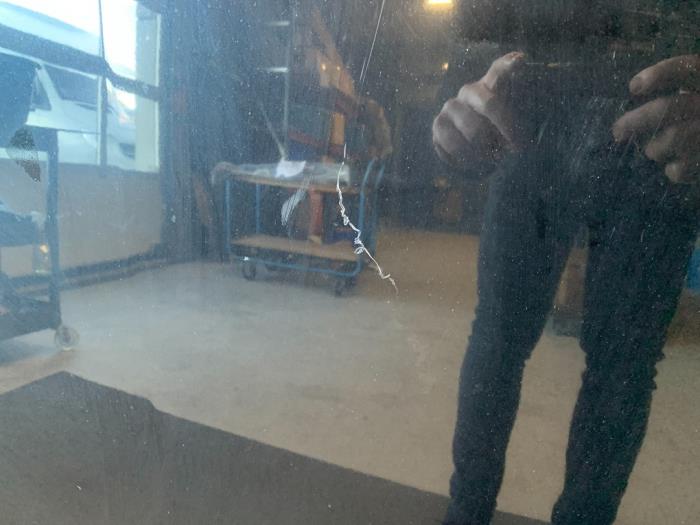In this photograph, a white Caucasian individual is depicted capturing an image of themselves in a mirror, their hands clasping a camera that obscures much of their body. The image has a slight blur, adding a sense of mystery. The person appears to be wearing black pants. Central to the composition is a prominent white line, likely a reflection from the mirror or screen that bisects the scene. The floor initially shows a brown carpet, transitioning to a grayish-brown surface further back.

In the background, a blue cart equipped with brown shelving and topped with a blue handle is visible, supported by wheels for mobility. To the left, an out-of-focus window frames the scene, showcasing a peculiar gray square positioned on its edge from the outside. Behind the cart, shelves cluttered with various boxes are discernible. Additionally, on the far left side of the image, there's a three-tiered gray cart also mounted on wheels, adding to the utilitarian feel of the setting. The overall ambiance suggests a practical, work-oriented environment with a mix of organizational elements.